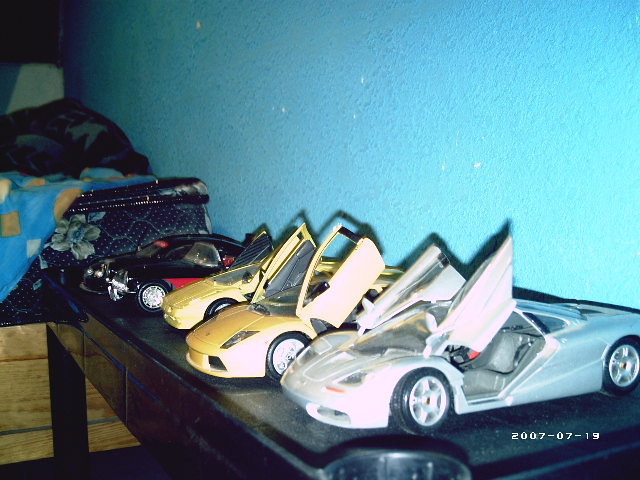This detailed snapshot features a collection of five model cars meticulously arranged on a sleek, shiny black table positioned against a pale blue wall. The table's surface catches the bright light shining directly on it, casting sharp shadows of the cars. The first car, a striking blue model, and the second, an identical futuristic yellow version, both have doors that open upwards like a DeLorean. The third, another yellow car, also appears to have futuristic features though it's hard to discern clearly. The fourth vehicle is a distinctive black convertible from the 1950s, accentuated with a red stripe around its edges. Completing the lineup is a sleek black sedan, possibly resembling a Jaguar, with all its doors closed. In the background, a faint piece of furniture, either a bed or a table, draped in blue, is barely visible. At the bottom right-hand corner of the photo, there's a date stamp reading "2007-07-19," anchoring the image in time.